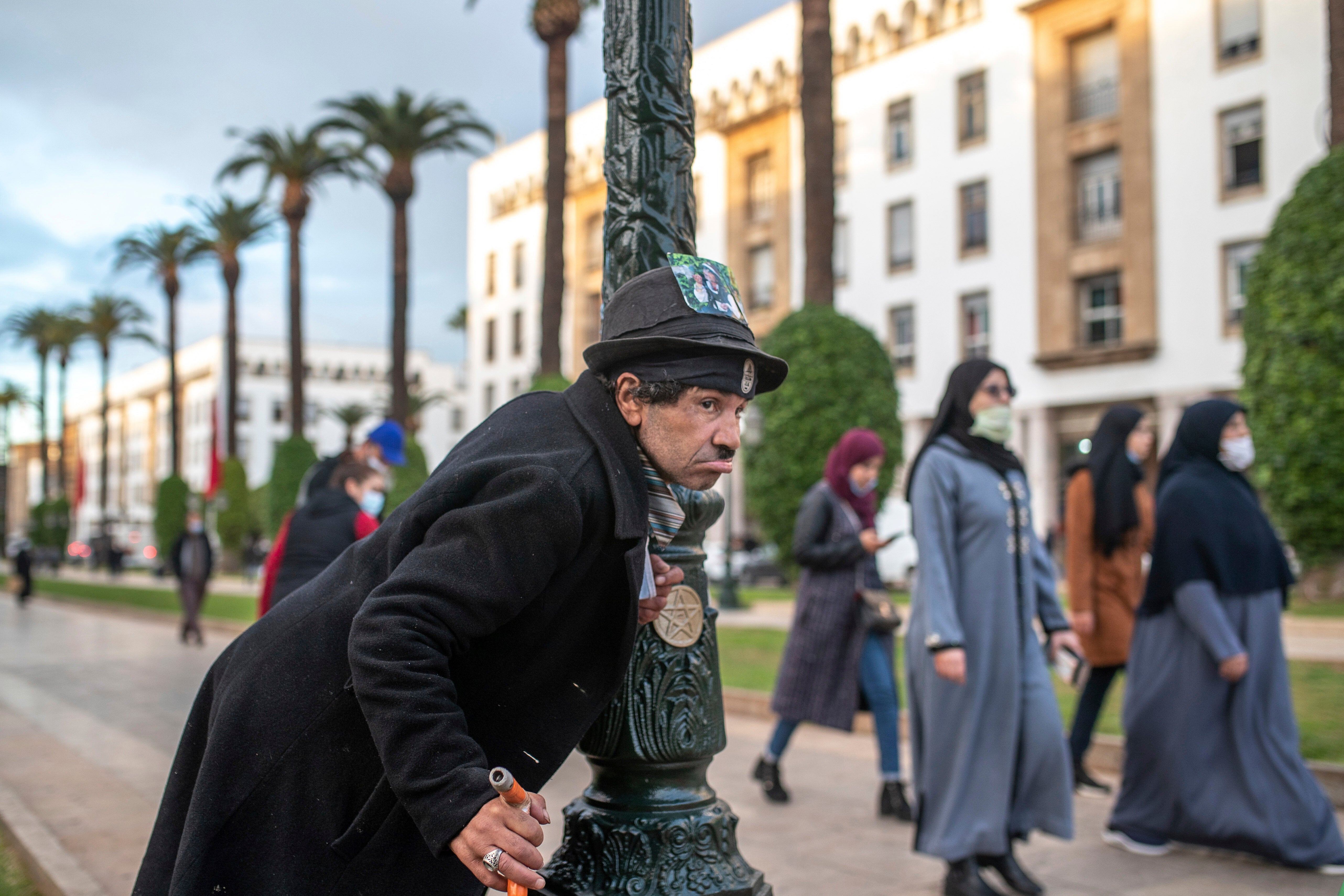In this street scene, a man is prominently positioned in the foreground, leaning against a dark green lamppost adorned with a Star of David. He has a somber expression, wearing a black fedora with a photo tucked into its band, and a long black wool trench coat. He clutches an orange object in one hand. Palm trees line the street, suggesting a tropical or warm climate. Behind him stands a large, elegant white and gold building. To his right, a group of women in hijabs and full-length robes are visible, some in black and one in burgundy, moving away from the man. Other figures blend into the background, with the street blurring into the distance.